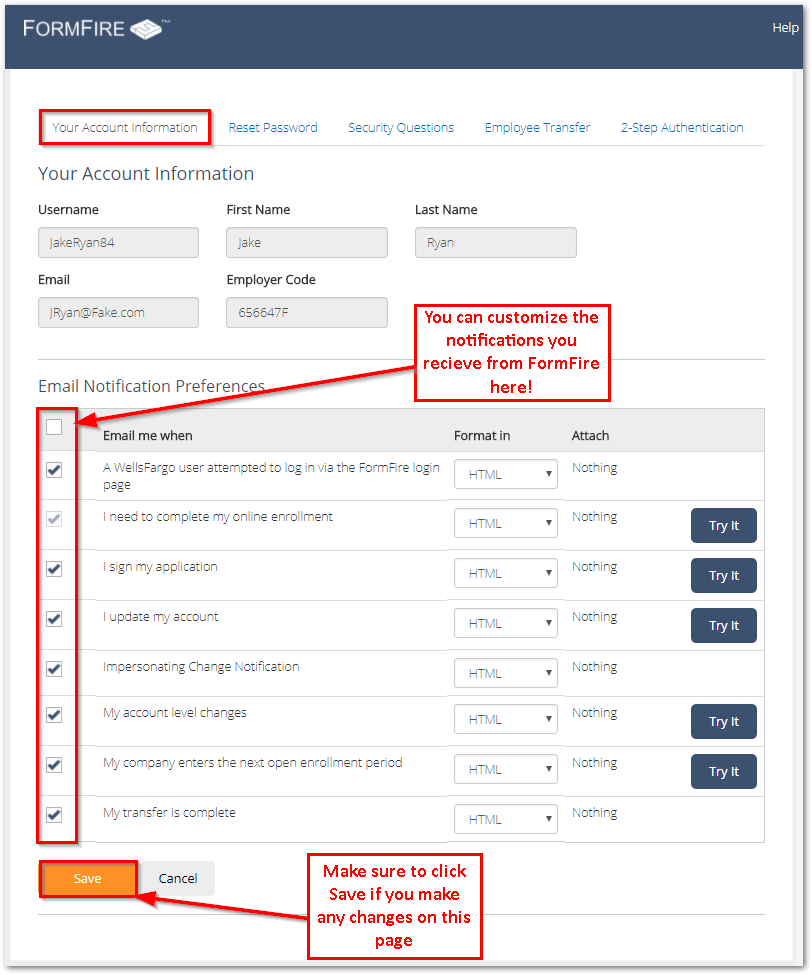**Detailed Caption for FormFire Account Settings Page**

The image depicts the Account Settings page on the FormFire website. The page is designed with a clear and structured layout:

- At the top left corner, the "FormFire" logo is prominently displayed, while the top right corner features a "Help" button for user assistance.
- Beneath the header, a navigational bar spans across the top, providing quick links to sections such as "Your Account Information," "Reset Password," "Security Questions," "Employee Transfer," and "Two-Step Authentication."

In the main content area, the "Your Account Information" section allows users to edit their personal details through input fields. These fields include:
- Username
- First Name
- Last Name
- Email
- Employer Code

Directly below these fields, there's a section titled "Email Notification Preferences." On the left side, several checkboxes are listed, each corresponding to different notification options. Some checkboxes are ticked, indicating active notifications, while others remain unticked. A red arrow emphasizes a customizable feature with the note, "You can customize the notifications you receive from FormFire here."

The notification options include:
1. *Email me when* a Wells Fargo user attempted to log in via the FormFire login page. (Ticked, format: HTML, attachment: None)
2. *I need to complete my online enrollment*. (Ticked, format: HTML, attachment: None, with a clickable "Try it" button)
3. *I signed my application*. (Ticked, format: HTML, attachment: None, with another "Try it" button)
4. *I update my account*. (Unticked, format: HTML, attachment: None, and a "Try it" button)
5. *Impersonating change notification* (Ticked, format: HTML, attachment: None)
6. *My account level changes* (Ticked, format: HTML, attachment: None, and a "Try it" button)
7. *My company enters the next open enrollment period* (Ticked, format: HTML, attachment: None, with a "Try it" button)
8. *My transfer is complete* (Ticked, format: HTML, attachment: None)

At the bottom of the page, a bold orange button with white text reads "Save," accompanied by a red arrow pointing to it, instructing users to click save if any changes are made. To the right of the "Save" button, there is an option to "Cancel" any edits.

Overall, this FormFire Account Settings page is comprehensive and user-centered, allowing users to efficiently manage their account details and notification preferences.